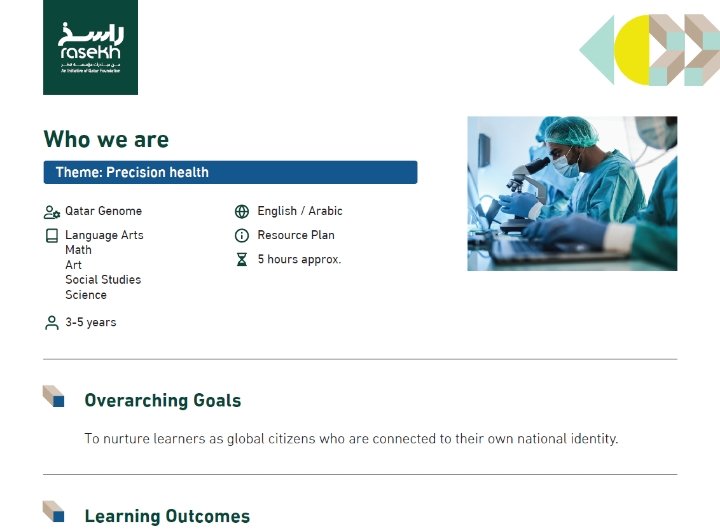The image features a green rectangular logo positioned in the upper left corner with the text "RASEKH" beneath it. Below the logo, in black font, is the phrase "Who We Are." A thin blue bar follows, displaying the words "Theme: Precision Health" in white font. Underneath the bar are the terms "Greater Genome," along with a list of subjects: "Language Arts, Math, Art, Social Studies, Science." This section is labeled as "Three to Five Years." 

To the right of the blue bar, there is additional text stating "English Arabic Resource Plan, Approx. Five Hours." Adjacent to this text is an image of doctors, dressed in blue smocks, hairnets, and blue gloves, intently examining specimens through a microscope. They are oriented towards the left side of the image.